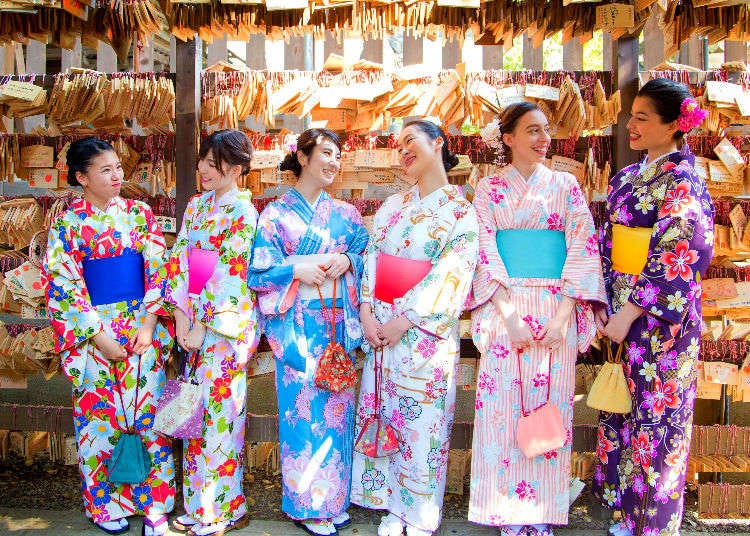The photograph features six women of varying heights and ages, likely between their 20s and late 30s, all of Asian descent, dressed in a vivid array of colorful kimonos adorned with intricate floral patterns. They stand side by side against a backdrop that appears to be part of a Japanese shrine, characterized by numerous wooden tablets inscribed with Japanese writing hanging above and around them. The image, though a bit blurry, captures each woman holding different colored purses and smiling warmly at each other, except for the one on the far left who has her mouth closed. The first woman wears a white kimono with red, blue, and pink flowers paired with a dark blue belt. The second woman also wears a white kimono embellished with red, yellow, and pink flowers and a dark pink belt. The third woman is in a predominantly blue kimono with pink flowers, matched with a white belt. The fourth wears a white kimono featuring a mix of colorful flowers and a light pink belt. The fifth woman's kimono is white with pink stripes and darker pink flowers, complemented by a light blue belt. The woman on the far right wears a purple kimono decorated with dark and light pink flowers, accented with blue and white blooms, and her outfit is completed by a yellow belt. Despite the varied details of their kimonos, the women's coordinated traditional attire and their joyful expressions convey a sense of unity and celebration.